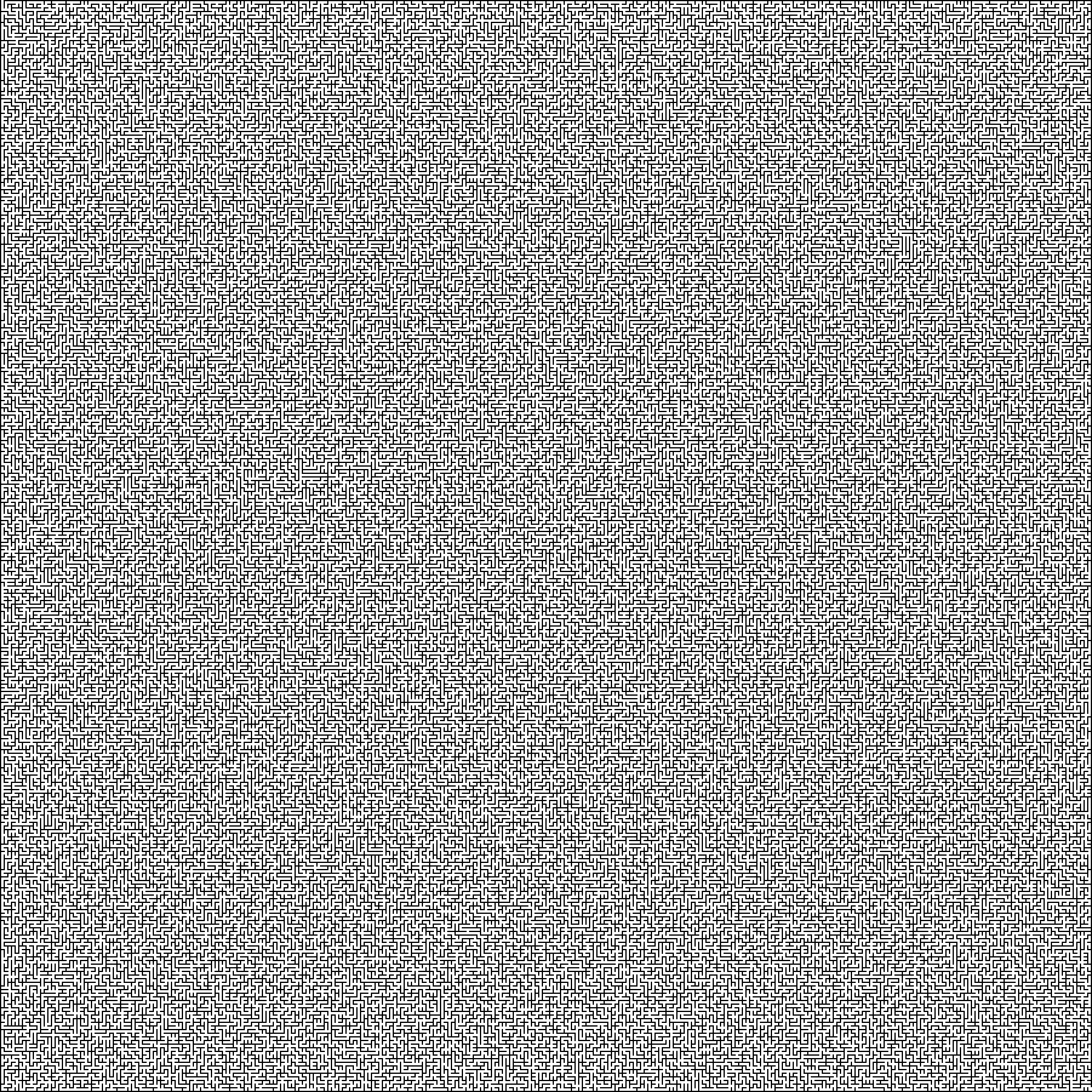The image is a black-and-white photograph featuring a large square with a white background. Within this square are extremely tiny black lines, intricately arranged to form what appears to be a maze-like pattern. From a distance, these densely packed lines create an effect reminiscent of television static, making the image look uniformly textured. However, upon closer inspection, one can discern the fine, maze-like quality of these lines. The patterns are so detailed and intricate that it's challenging to follow any distinct maze path, if one even exists. The overall effect is a fascinating blend of simplicity and complexity, combining the uniformity of static with the intricate detailing of a miniature maze. This unique interplay between distance and detail defines the entire photo.